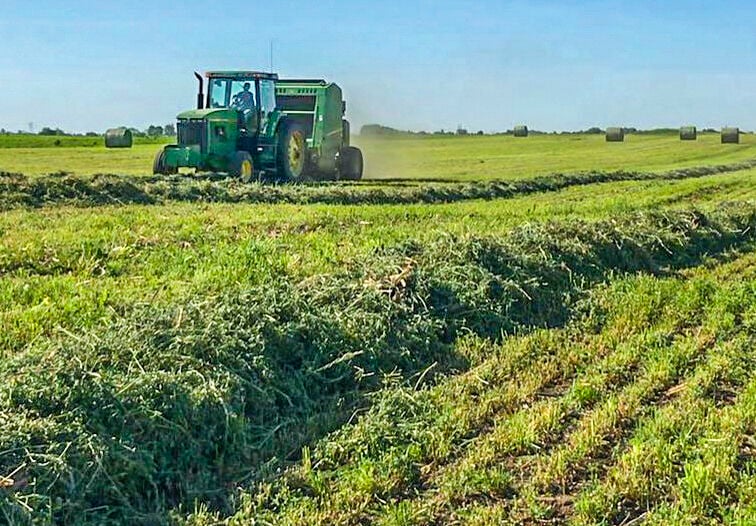The image captures a bustling agricultural scene on a farm during a round hay baling operation. At the forefront, a large green John Deere tractor, equipped with yellow wheels and an enclosed cab, is meticulously plowing through a vast green field. The tractor is pulling a round baler, and the driver is visible within the glass-enclosed cab, operating the machinery. The field is primarily covered in grass, which has been methodically cut and raked into neat rows, save for a few bunched-up patches that stand taller. In the background, numerous round hay bales, already formed, are scattered across the landscape. The sky above is a soft blue, tinged with a slight gray haze near the horizon, setting a tranquil daytime scene. Dust trails can be seen emanating from the back of the baler, accentuating the active nature of the farm work.